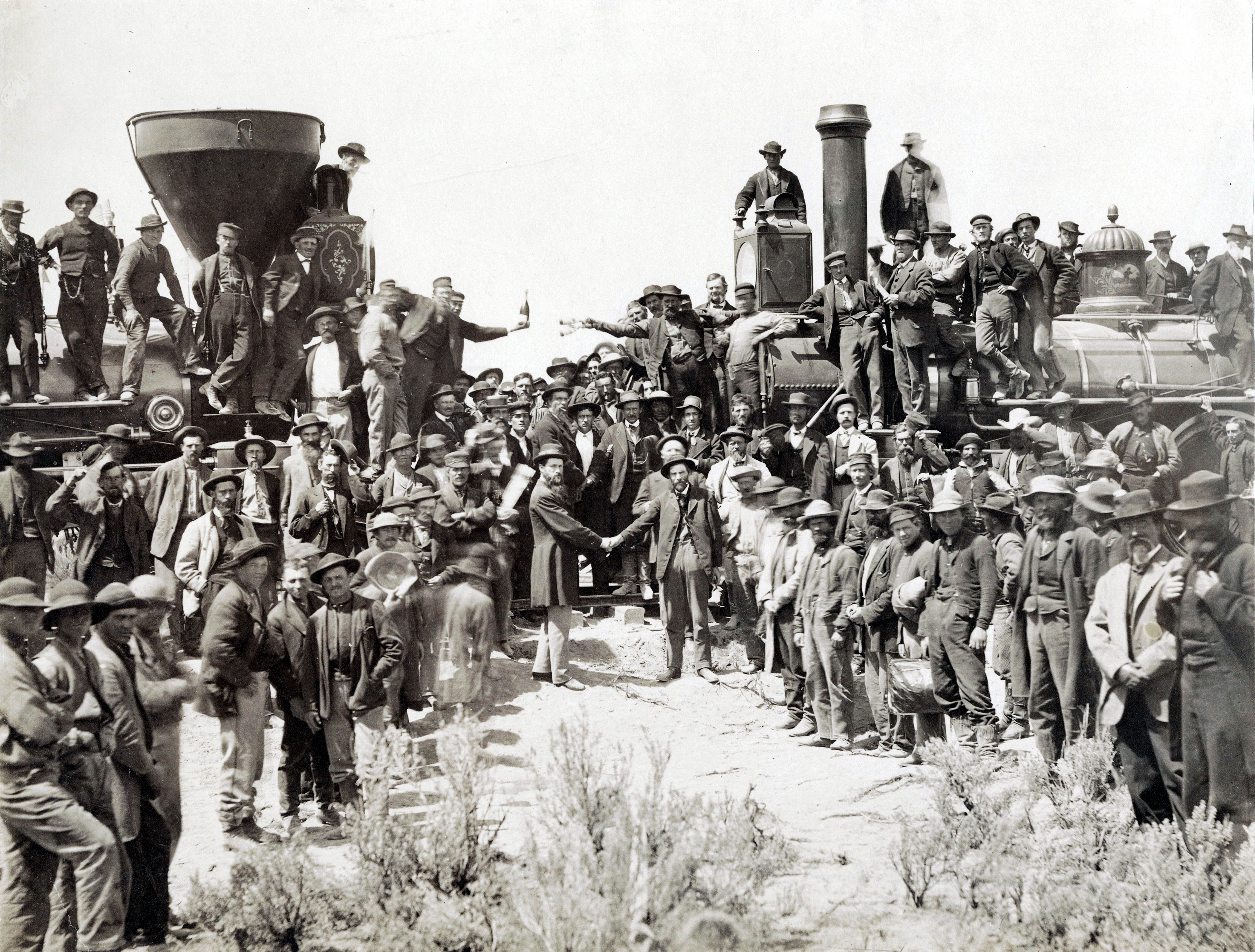A mid-1800s black-and-white photograph captures a historic moment where two steam locomotive engines meet face-to-face on parallel train tracks in a desert landscape. The scene is bustling with hundreds of men, presumably railroad workers, who are dressed in suits, fedoras, and hats, conveying a sense of accomplishment and camaraderie. Many of them are posing for the camera—some standing on the locomotives, others in front, beside, or atop of the engines. Prominent in the middle are two individuals shaking hands, symbolizing the successful connection of the rail lines built from opposing directions. In the background, one man holds a bottle of champagne while another holds out a glass, suggesting a celebratory mood. The bottom of the image shows more workers, some appearing to stand on an object with a trophy-like structure behind them. Brushy plants, indicative of a desert setting, line the base of the picture, further emphasizing the rugged environment in which this monumental achievement took place.